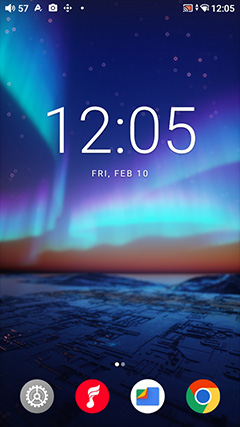The image depicts a smartphone screen displaying a lush and vibrant screen saver. The lower portion of the screen showcases a captivating view of Earth, with the planet's curvature adorned by luminous aurora lights that gracefully curve above it. The top of the screen opens up to the vast, dark expanse of space speckled with twinkling stars. The color palette consists of deep blues, purples, and aqua tones, creating a mesmerizing and aesthetically pleasing background.

Prominently displayed in large white font at the center of the screen is the time, "12:05," with the date "Friday, February 10th" written in a smaller font just below. At the very bottom, there are four clickable tabs: Google, Settings, a red tab with a mysterious white swirly design, and a white tab featuring an icon that looks like folded paper, possibly representing an email app.

In the upper-right corner of the screen, the time "2:05" is shown once again, along with the Wi-Fi signal icon. On the upper-left side, there is an icon of a camera, and the volume is indicated to be at 57%. The overall design is vibrant and detailed, providing an informative yet visually engaging experience.